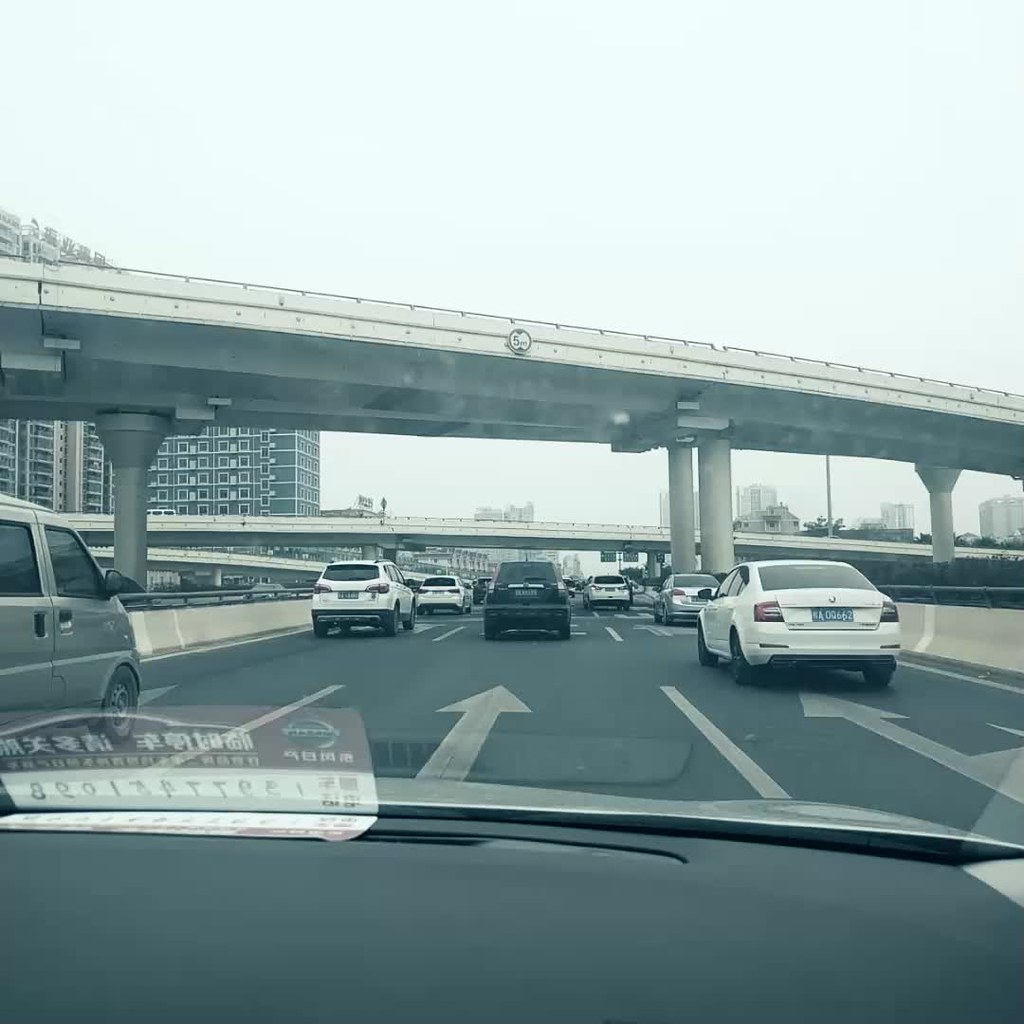This photograph, captured from the passenger seat of a car, presents a dynamic and detailed view of an active highway. Inside the car, part of the dashboard is visible, accented by reflections that include the prominent Nissan logo and an array of numbers and Asian characters, likely Chinese or Japanese. The highway itself is marked with clear directional arrows, indicating that the traffic is moving in one direction. To the right, an additional lane offers an option to either continue straight or turn right, suggesting a potential turning lane. 

On the road, a grey van is positioned beside the car from which the photo was taken. In the lane to the left, there is a white SUV followed by another white SUV in front. Directly ahead, a black SUV leads the traffic flow. In the far right lane, two sedans, either white or silver, are visible. Adding to the urban landscape, a road bridge spans across the highway, with several buildings rising in the background, contributing to the bustling scene.